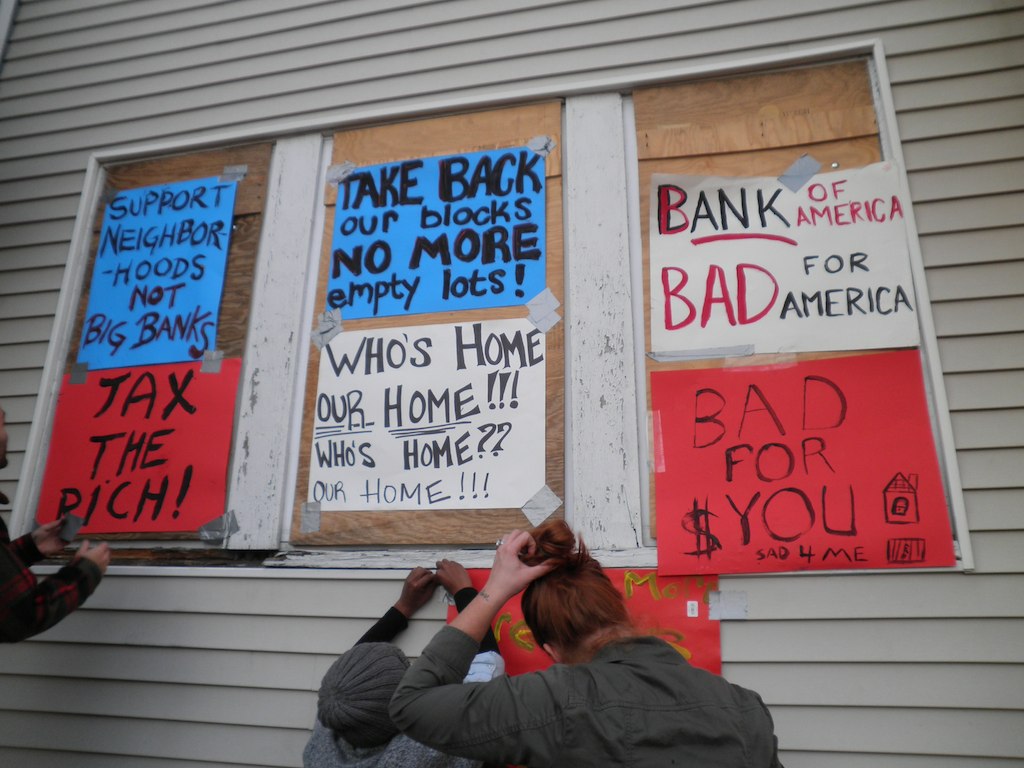The image depicts a group of people hanging protest signs on the boarded-up windows of a residential building with gray slats. The signs cover the windows and collectively criticize large banks. Starting from the left, the signs read: "Support Neighborhoods, Not Big Banks," "Tax the Rich," "Take Back Our Blocks, No More Empty Lots," and twice, "Whose Home? Our Home." On the right side are the messages: "Bank of America, Bad for America," and "Bad for You - Sad for Me." Below these, another sign is being put up but is obstructed by two individuals. One person, wearing a hat with a white t-shirt over a black long-sleeve shirt, is applying gray duct tape to the "Tax the Rich" sign. A second individual, with reddish hair in a bun and a gray long-sleeve shirt, is scratching the back of her head. Their faces are not visible in the image.